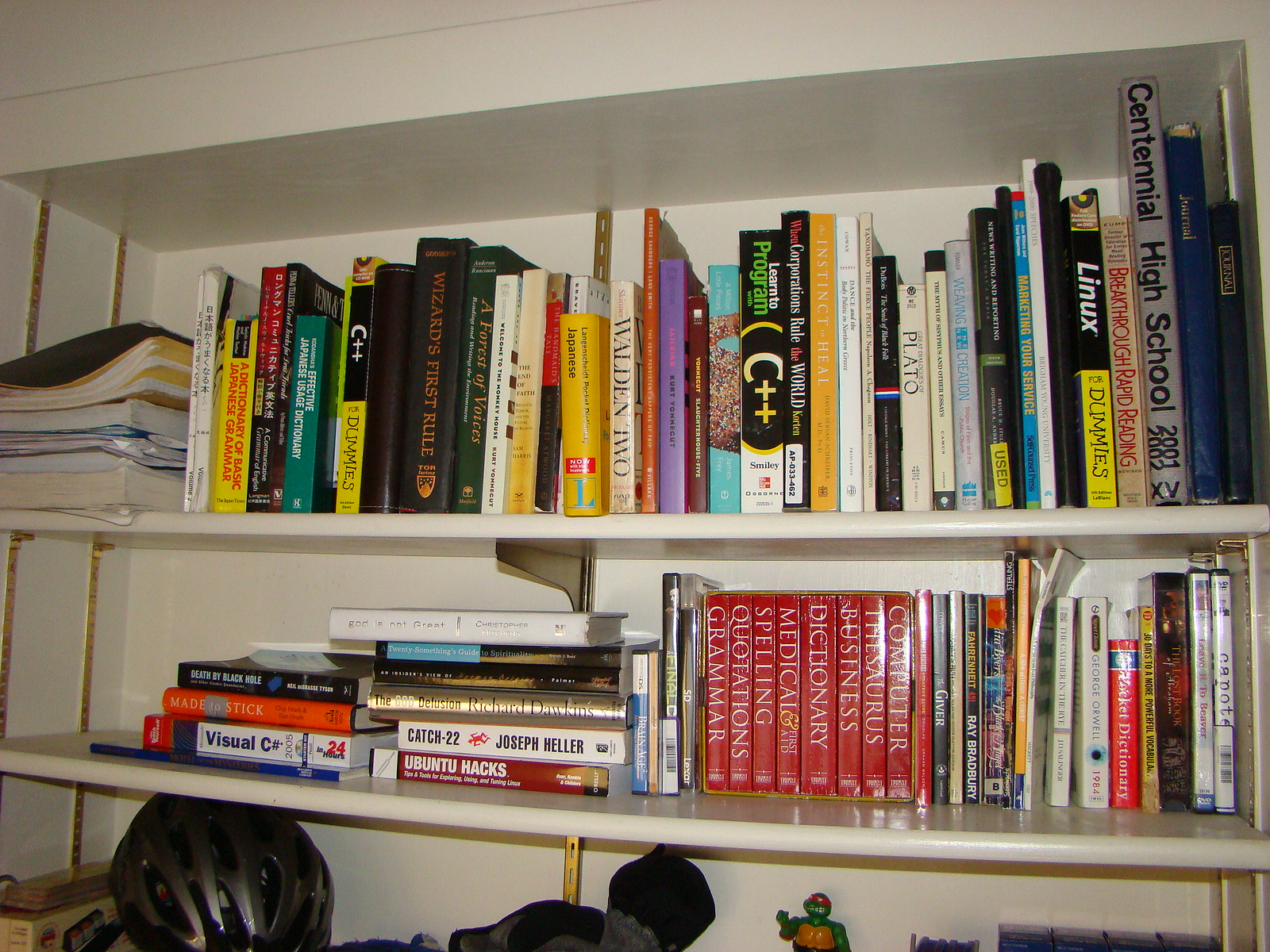This image depicts a detailed view of a white bookshelf, positioned in what appears to be a bedroom. The bookshelf features two distinct shelves, each filled with a variety of books. 

On the top shelf, most books are neatly stacked vertically, while a few on the left-hand side lay horizontally. The collection comprises a diverse mix of literature, including computer programming guides, a book on learning Japanese, texts on Japanese grammar, resources for learning Linux, and even a high school yearbook. The covers of these books display an array of colors, including blue, yellow, white, and green.

The lower shelf also holds an assortment of books, some lying flat and others standing upright. Notable titles include a Visual C++ reference book, the novel "Catch-22," an array of learning books, a dictionary, a computer thesaurus, and a cookbook. 

Below these shelves, a few other personal items are visible. Among them is a bicycle helmet and a small part of a Teenage Mutant Ninja Turtle figure, adding a touch of personality to the scene. 

The bookshelf is characterized by its white finish and gold hinges. The absence of people in the photograph lends it a quiet, contemplative atmosphere, capturing a slice of everyday life in a typical bedroom setting.